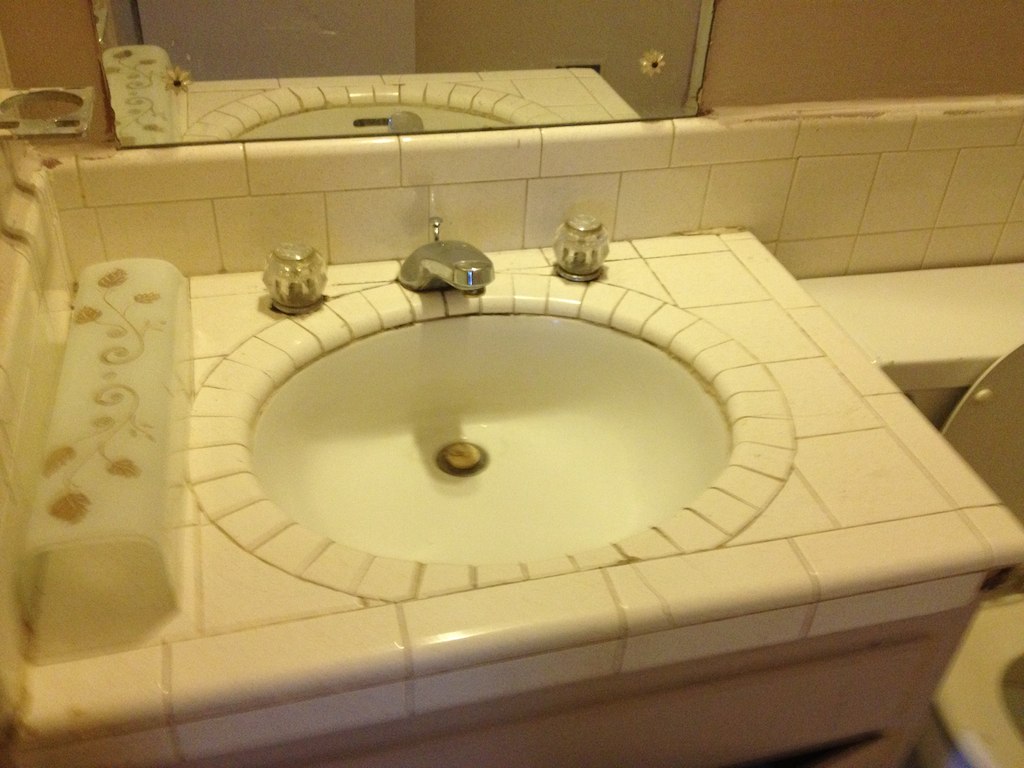This image depicts a detailed view of a white bathroom sink set against a backdrop of white and beige tiles. The sink, centrally positioned, is crafted from square white tiles, which show dark brown cracks in the grout lines. Surrounding the pure white interior of the sink is a tiled structure adorned with small, white ridges and tiles. In the center of the bowl, there is a metallic, steel drain, offset by a small gold knob. The faucet and the two clear, circular glass handles, arranged for hot and cold water, add a touch of elegance with their chrome finish.

Above the sink, there is a mirror affixed to the wall, which provides a reflection of the well-lit interior, suggesting the presence of an overhead lamp, though the actual lamp is not visible. To the left of the sink, a ring designed to hold toothbrushes is mounted on the beige-hued wall, contributing to the functionality of the space. Additionally, the right side of the image captures a glimpse of a white toilet, its cover up and seat down, completing this intimate portrayal of a somewhat aged, yet charming bathroom corner. The close-up view also reveals some scuffs and minor breakages, indicating wear over time.